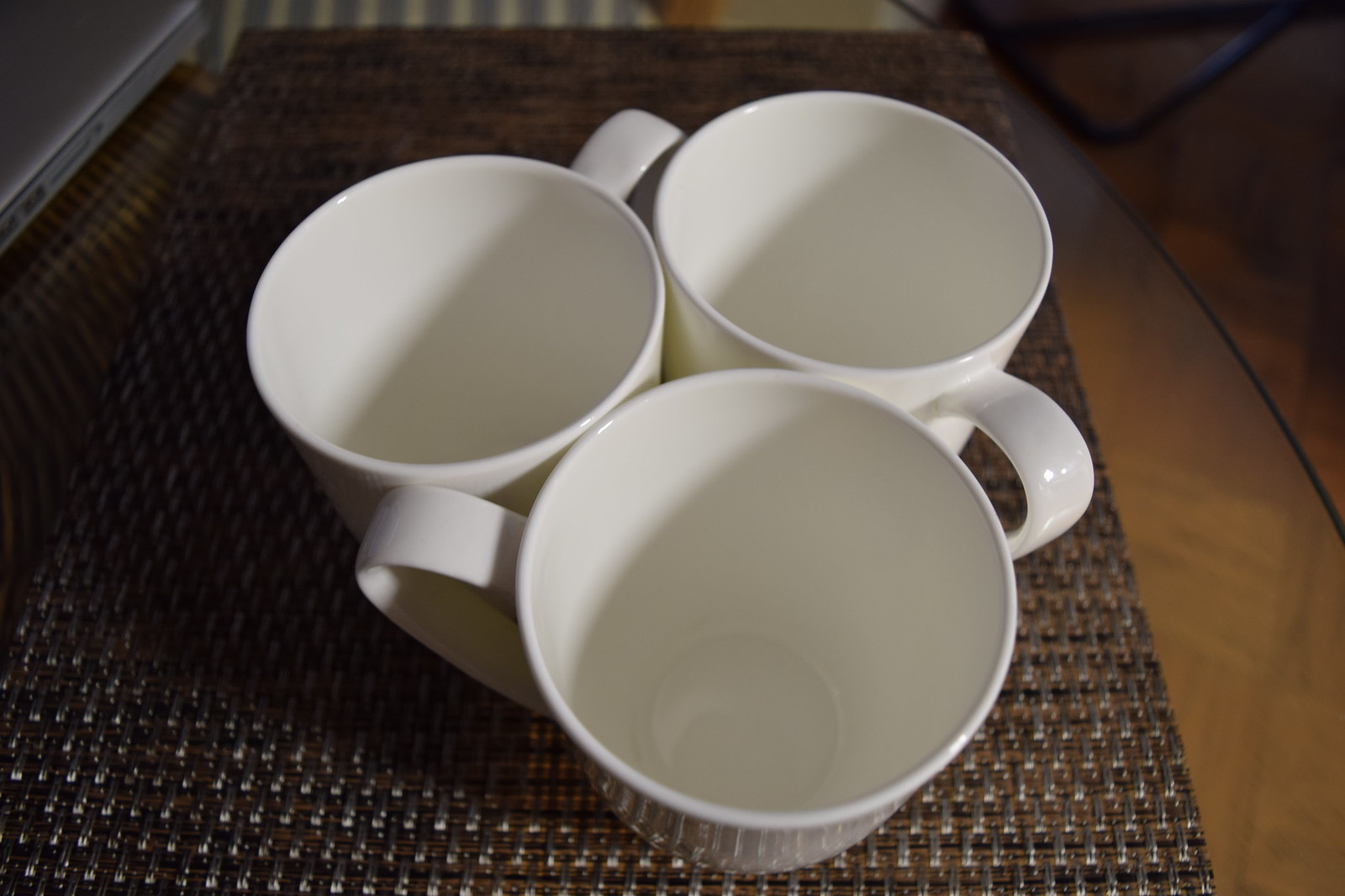This color photograph, taken indoors in a dimly-lit room, depicts three plain white porcelain coffee mugs arranged artfully in an upside-down triangular pattern on a dark brown woven placemat, which rests on a wooden table. The mugs are empty and feature smooth, curved handles that resemble flat, curved strips of pasta. Their handles are positioned so that each one touches the next, forming a cohesive circular arrangement. Shot slightly from above, the composition captures the subtle highlights on the woven mat and the clean, minimalist design of the mugs. At the upper edge of the photograph, a glimpse of a blue and white striped fabric—likely part of a chair—is visible. Additionally, in the upper left corner, there is a silver metallic object that looks like a VCR. The background hints at a green wall with white trim. The table also has a black element, possibly a piece of wire, visible on the right side.